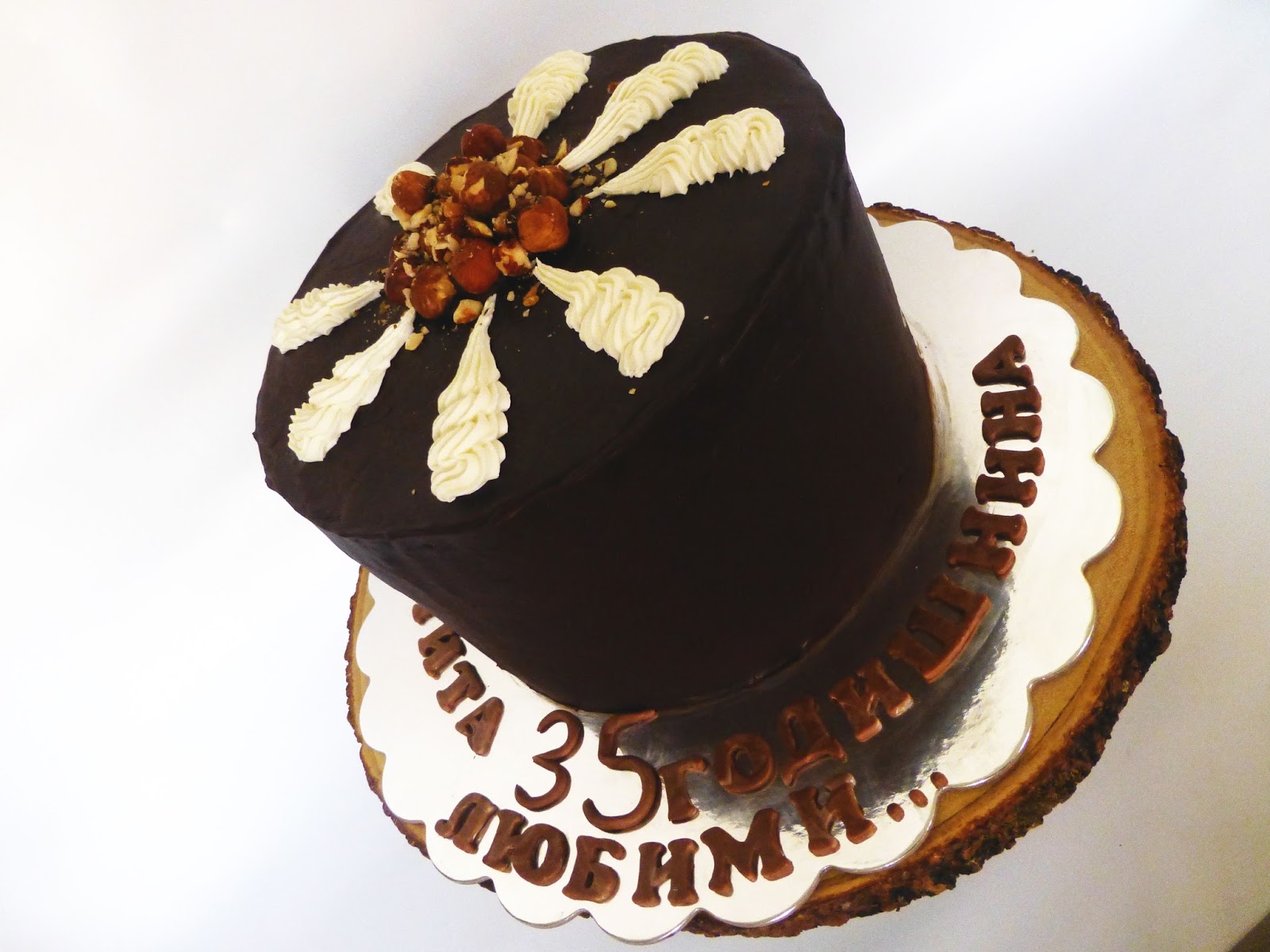This color photograph depicts a decadent chocolate cake positioned on a white table. The cake, bathed in dark chocolate icing, is further adorned with white cream piping on its top surface, arranged in a pattern that resembles eight balloon shapes. In the center, a generous mound of hazelnuts adds to the cake's rich texture. The entire ensemble rests on a wooden platter, which appears to be a thin, tan-colored slice of a tree, complete with bark around its edges. Beneath the cake is a decorative silver placemat featuring a chocolate inscription, which includes the numbers "35." This detail, along with the ornate presentation, suggests that the cake is likely intended for a 35th birthday or anniversary celebration.